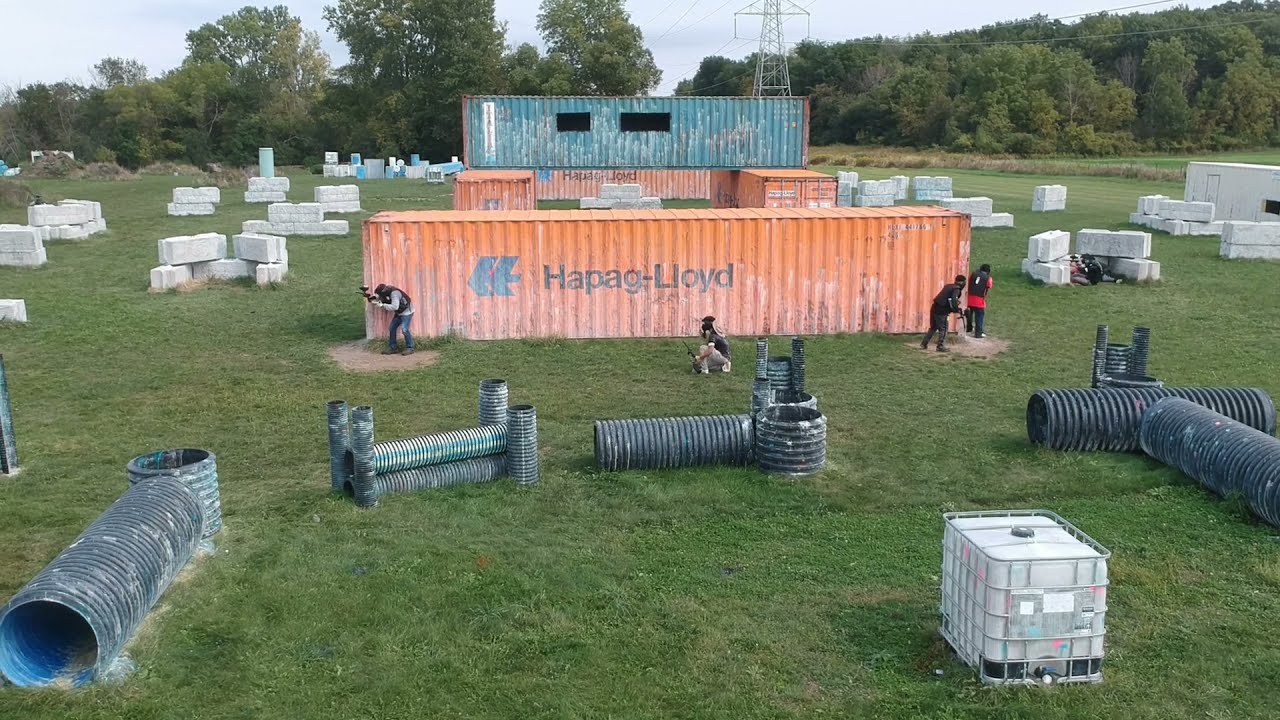The photograph captures a vivid and detailed scene of a wide-open, grassy field under bright daylight. Dominating the center of the image is a large, beat-up yellow shipping container with a blue logo and the words "Hapag-Lloyd" written in black font. Closer to the viewer, partially hidden behind this container, are four individuals dressed in dark colors, armed with paintball guns. Scattered in the foreground are structures made of large black tubes and pipes, covered in paint and debris. 

The field itself is a lush green, with patches of bright green grass stretching out into the distance, where copses of vibrant trees can be seen. Other shipping containers are visible further back; one is an orange "Hapag-Lloyd" container, similar to the one in the foreground, with a blue container stacked atop it, marked by two dark windows. Additional white stone structures are randomly scattered around the field, adding to the sense of organized chaos within the space. Overhead, power lines stretch across the top right-hand corner of the image, adding an industrial element to the otherwise natural landscape.